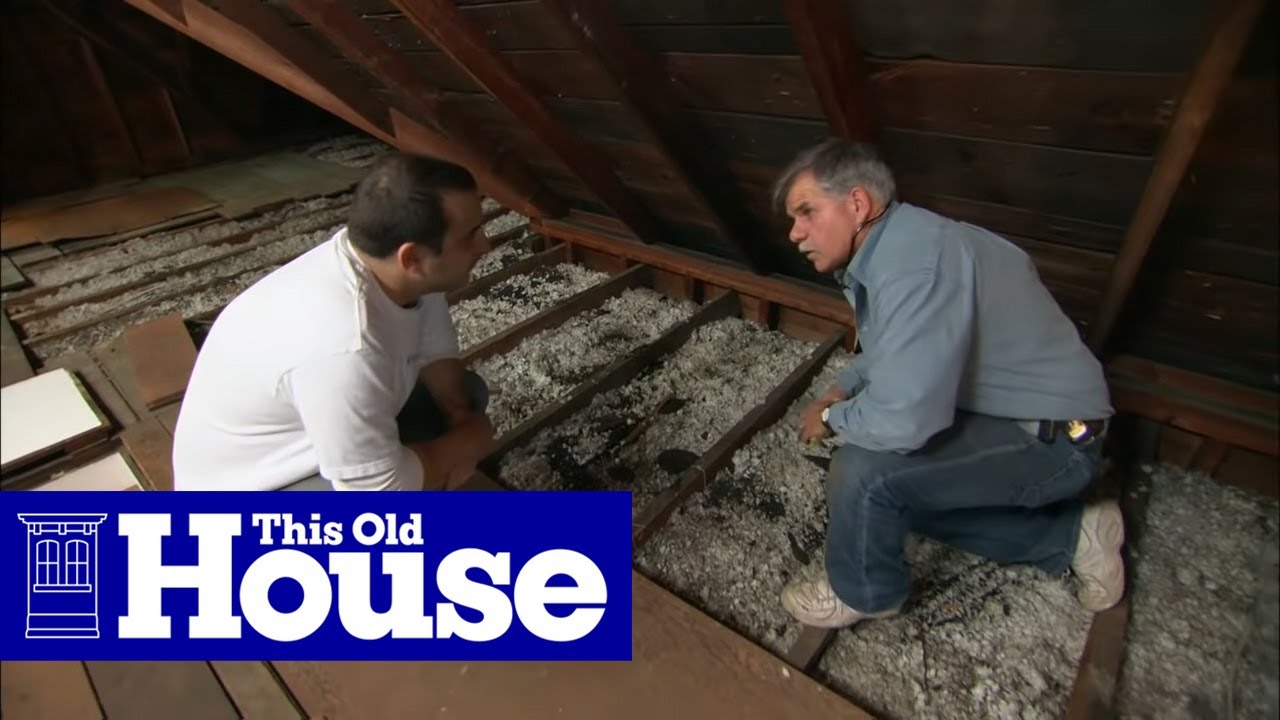In this landscape-oriented still shot from "This Old House," we see a detailed scene set in an attic. The image features Tom Silva, a recognizable host of the show, alongside the homeowner. Tom Silva, dressed in a blue shirt, denim jeans, and white tennis shoes, is perched atop a couple of rafters, examining the insulation between them. Meanwhile, the homeowner, clad in a white shirt, is crouched on a section of the attic floor that is decked with boards. The open hatch of the attic entryway is visible behind him. The background includes a large blue text box featuring the iconic "This Old House" logo with a small house icon. The setting suggests that the men are deep in conversation, likely discussing the condition and possible repairs of the attic insulation or the wooden structures. Dust and debris are scattered around, indicative of the ongoing work or assessment in progress.